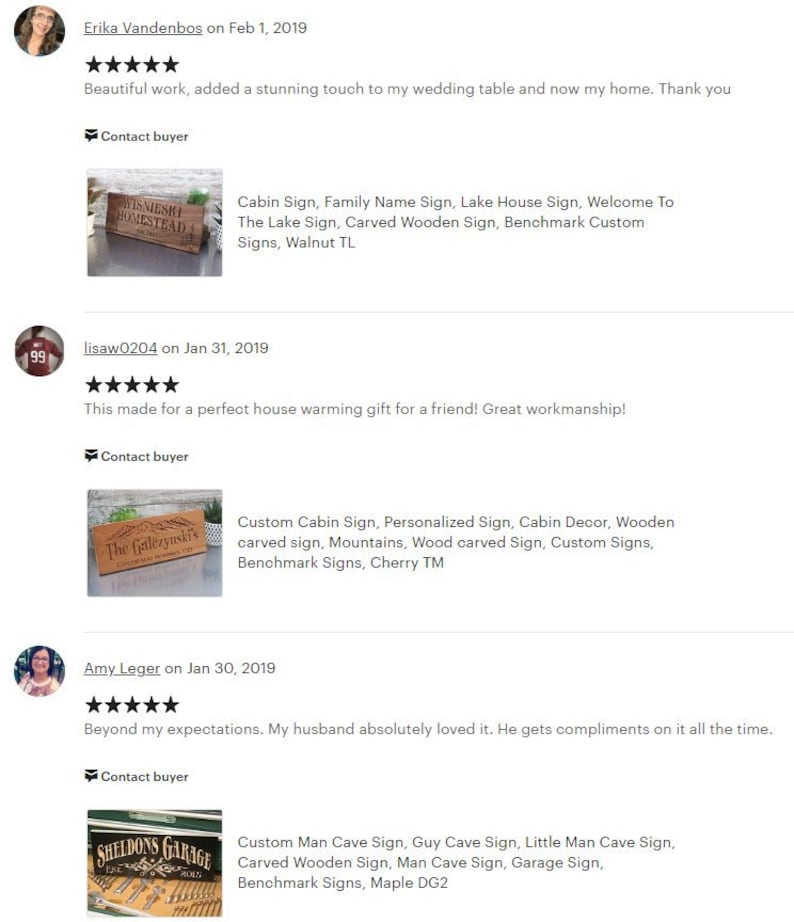The image features a review compilation of various wooden signs, showcasing detailed feedback from multiple customers:

1. **Erica Vanna Boasts - February 1st, 2019**
   - *Rating:* 5 out of 5 stars
   - *Review:* Erica praised the sign for its beautiful workmanship, stating it added a stunning touch to the wedding table at her home.
   - *Product Description:* A carved wood sign reading "Wisdom Wisniewski Homestead." To the right of the sign, it's labeled under different categories: Cabin Sign, Family Name Sign, Lake House Sign, and Welcome to the Lake Sign.

2. **Lisa AW - January 31st, 2019**
   - *Rating:* 5 out of 5 stars
   - *Review:* Lisa mentioned that the sign made a perfect housewarming gift.
   - *Visual Description:* The reviewer, wearing a red soccer jersey, is depicted alongside the review.

3. **Amy Leger - January 30th, 2019**
   - *Visual Description:* A wooden sign labeled "Sheldon's Garage" with a burned effect. The sign features a series of tools in front of it and includes labels such as Custom Man Cave Sign and Little Man Cave Sign, indicating its purpose as personalized décor for a man cave.

Each review is accompanied by the review date, a brief description of the sign, and a visual snippet of the wooden signs they had custom-made, including images of the reviewers and their contexts.